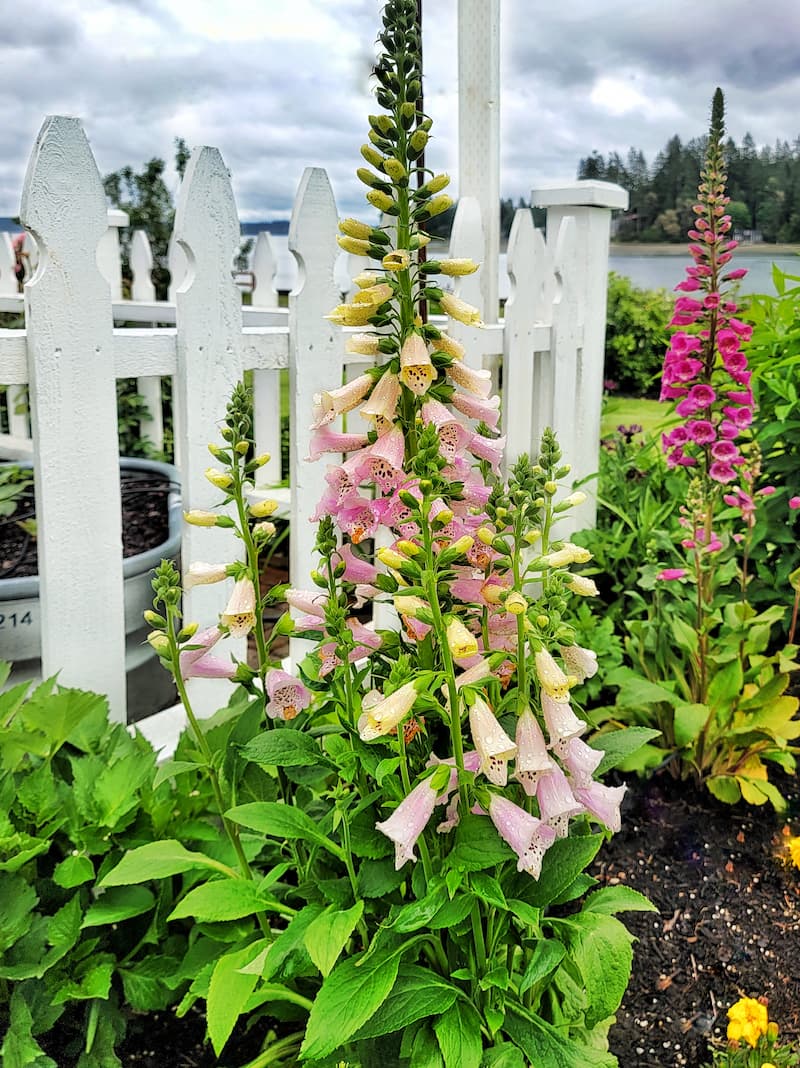The vertical rectangular photograph captures a serene outdoor garden scene framed by a white picket fence that borders a patio. Inside the fence, a silver planter holds a plant amidst dark, rich soil. The sky above is overcast with heavy gray clouds, suggesting a calm, cloudy day. Tall green trees and a glimmer of a body of water, likely a pond or lake, are visible in the distant background.

Outside the fence, the main focus of the image is a variety of tall flowering plants growing robustly from the black soil. Prominently featured in the foreground is a Christmas tree-shaped plant adorned with pink blossoms that rise halfway up its sturdy stalk, surrounded by lush green leaves at the base. Further back at the corner of the fence, another similar plant with darker pink flowers climbs three-quarters of the way up its stem, indicating it is not as tall. Other plants with green stems showcase yellow and light yellow bulbs that hint at imminent blooming. The scene blends the blooms and the natural backdrop into a picturesque and harmonious garden oasis.